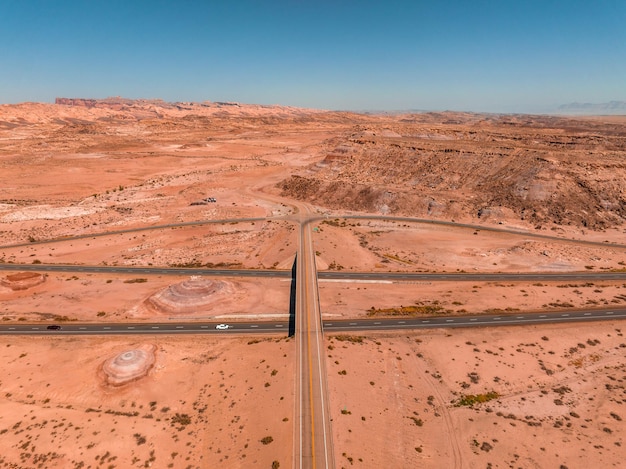This aerial photo captures a stark desert landscape, likely situated in the southwestern United States, such as New Mexico or Arizona. The land is covered in hues of oranges, peaches, and medium browns, resembling red clay or sand. The scene is devoid of vegetation, with no trees in sight and featuring some rocky, plateau-like formations in the distance.

The photo showcases a complex network of roads carving through the barren terrain. Two parallel highways run horizontally across the image, approximately cutting through the center. Each highway has two lanes, and they stretch left to right across the frame. In the foreground, you can see a white vehicle and a dark car traveling towards the right.

A notable feature is the road that starts from the bottom center of the image, running vertically upwards. This road intersects the horizontal highways and continues up slightly more than halfway before splitting into two branches that veer diagonally downwards, forming an angular shape that resembles a dragonfly. The upper portion of the image is a clear blue sky dotted with patches of white fog-like clouds, offering a stark contrast to the earthy tones beneath.